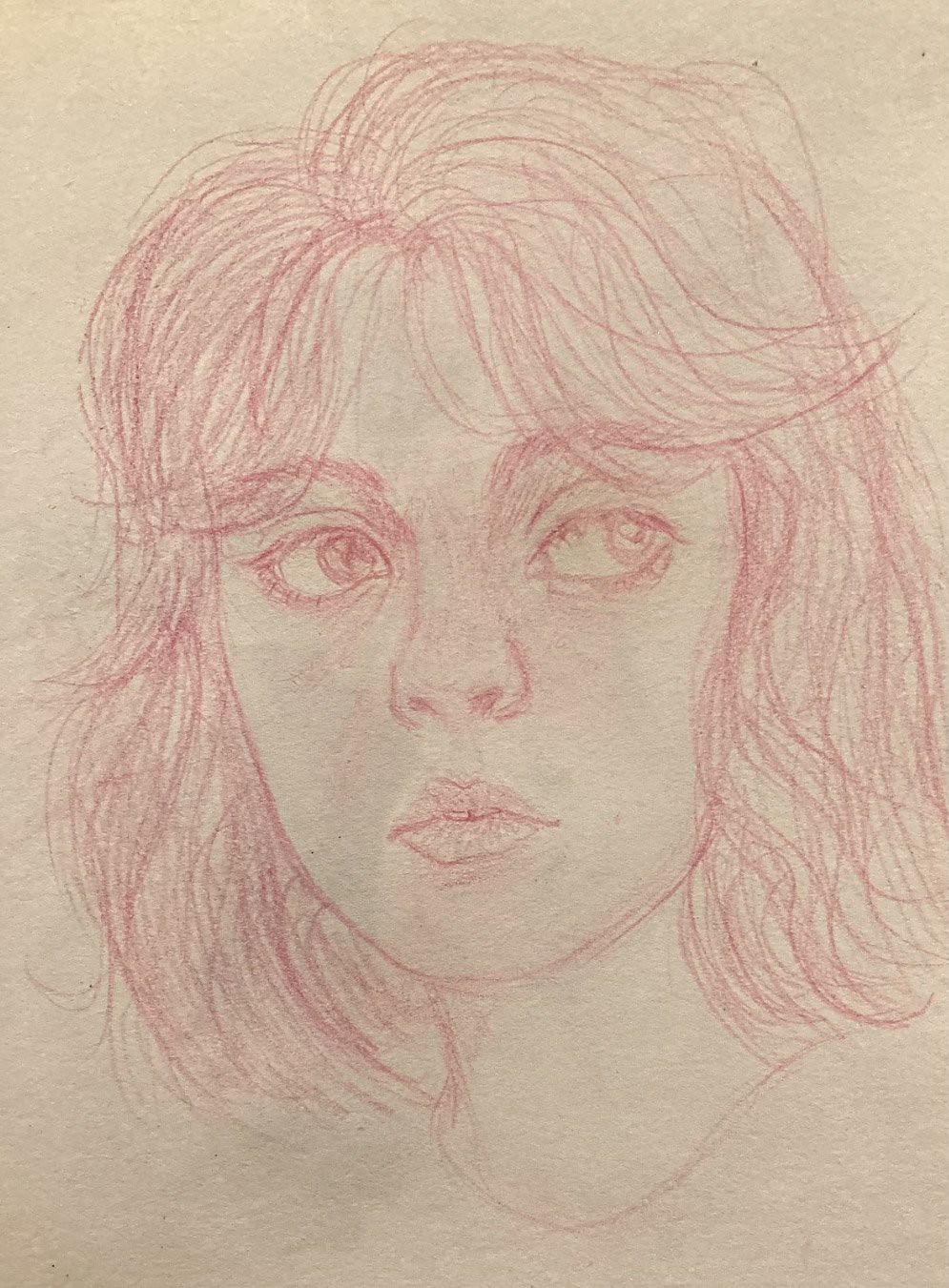This image is a detailed sketch of a woman or older teen, created on cream-colored, textured drawing paper with a pinkish-red colored pencil or pen. The artwork captures her shoulder-length, wavy hair that falls in sweeping bangs, rendering a wispy appearance that frames her face and covers her ears. The woman has a contemplative, wistful expression, with her full lips closed and slightly pursed, revealing the tip of two teeth. Her eyes, large and distinctively lighter due to the shading, gaze thoughtfully to the left, conveying a deep sense of introspection and mild concern. Her prominent eyebrows further define her expressive face. Despite being a rough sketch, the drawing is notably well-executed, focusing on her featured characteristics and rendering them with considerable detail.